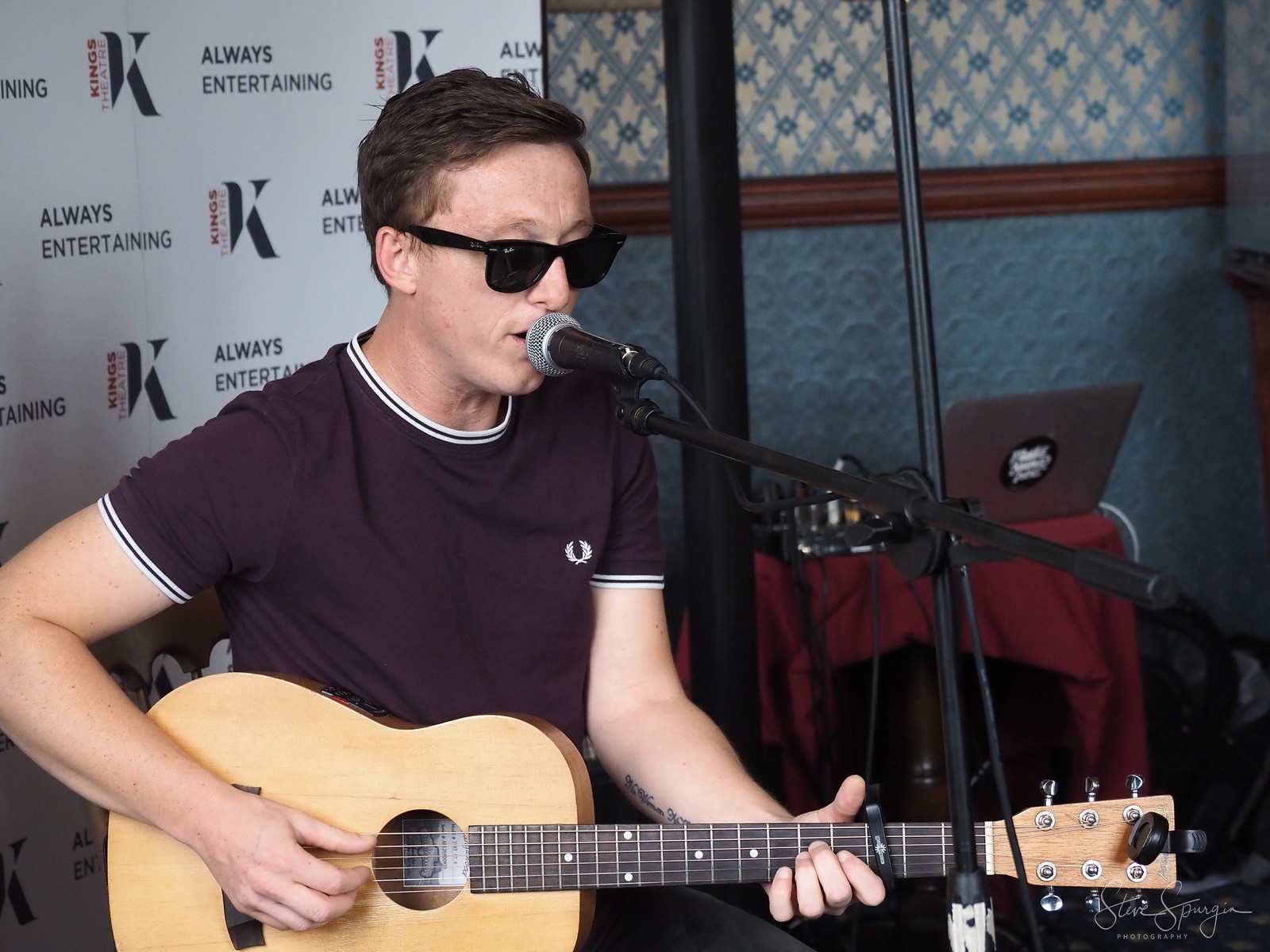The image captures a white male musician, likely in his 30s, sporting short brown hair and dark Ray-Ban sunglasses. He is seated, playing a light wood-colored acoustic guitar and singing into a microphone that is positioned right at his lips. He's clad in a black short-sleeved t-shirt with white accents on the collar and sleeve ends. Behind him, a prominent white backdrop features the repeated slogan "Always Entertaining" and the King's Theater logo, a stylized black letter "K" with the theater's name written vertically alongside it. The backdrop does not span the entire image; to the right, a small table draped in a burgundy red tablecloth hosts audio recording equipment, including an open laptop. This section of the background showcases a dusky blue fabric wallpaper interspersed with wooden trim and a patterned wallpaper adorned with white diamond shapes.